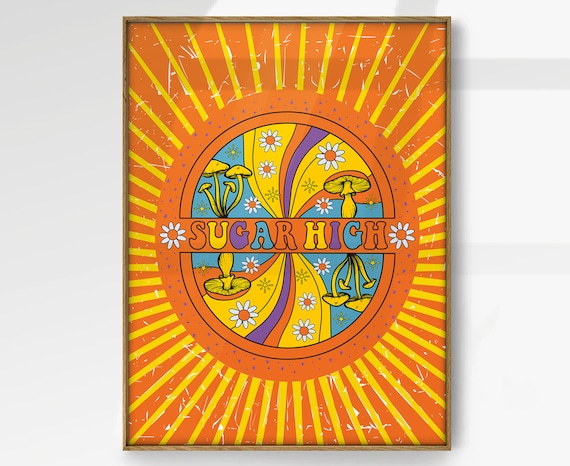This artwork, reminiscent of 1960s psychedelic style, features a vibrant composition of a multi-color print on a light gray background. The square piece has a thin brown border framing a vertically rectangular image. At its core is a central orange circle radiating bold yellow lines, mimicking the sun. The words "Sugar High" are boldly displayed in multiple colors—orange, yellow, purple, blue—across the center of the circle, captured in playful, bubblegum-style lettering.

The interior is divided into four sections, with each quadrant featuring vivid depictions of mushrooms and daisies. The mushrooms appear in an intriguing mirrored arrangement: the top section has mushrooms pointing upwards, while the lower section has them pointing downwards, with daisies interspersed among them. Surrounding the surreal center are swirling patterns of yellow, purple, and orange, enriching the piece with a dynamic, fabric-like impression that complements the overall trippy aesthetic. The entire composition embodies the essence of a '60s era sunshine scene, bursting with color and whimsical floral and fungal motifs.